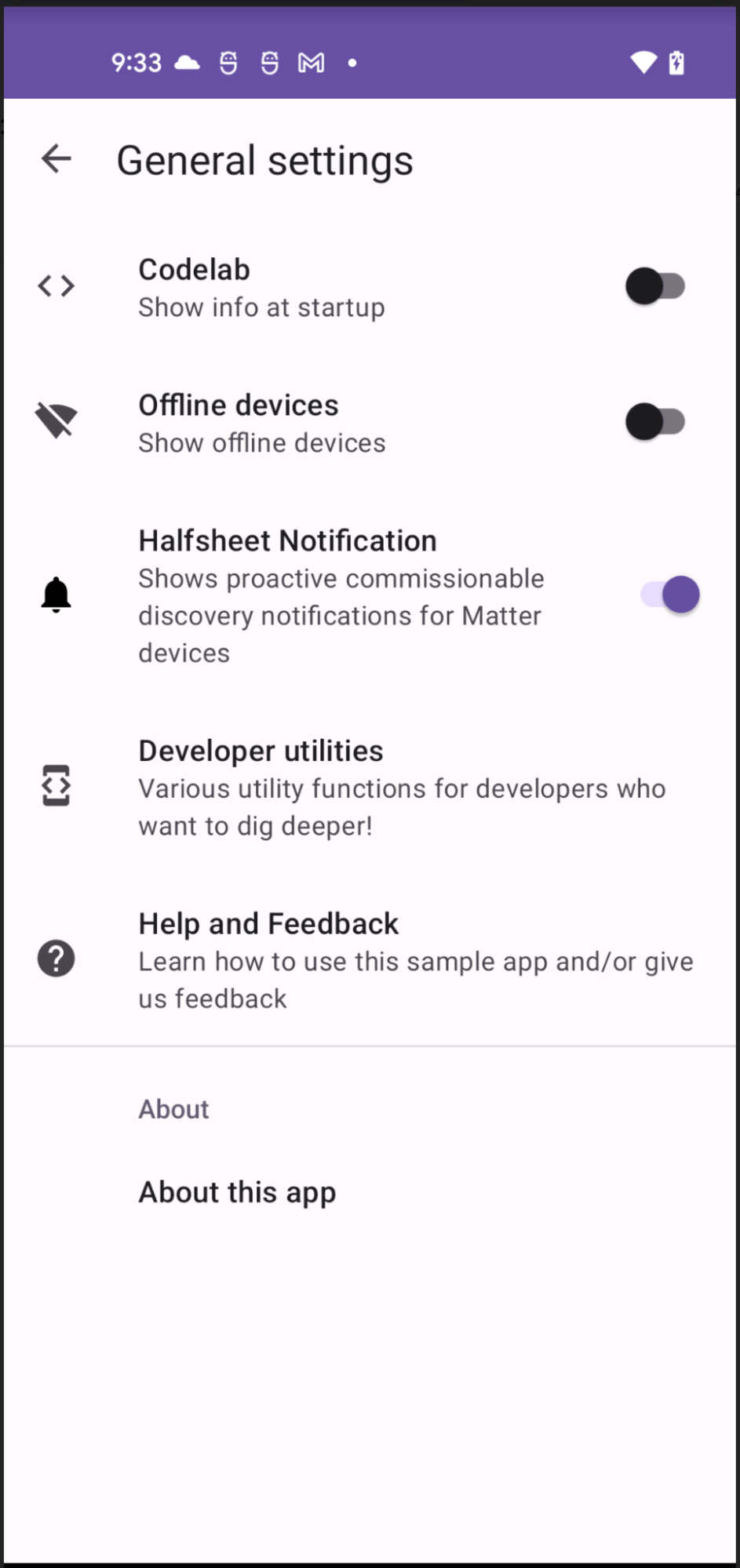This screenshot displays the settings screen of a mobile device. At the top, there's a purple status bar showing the current time and a battery icon. The main title on the screen reads "General Settings." Below this title, several settings options are listed, each accompanied by an on/off toggle switch to the right. The available options include "Codelab," "Offline Devices," "Half Sheet Notification," "Developer Utilities," and "Help and Feedback." Among these, only the "Half Sheet Notification" is toggled on, while the others are turned off. At the bottom of the screen, there is a clickable tab labeled "About This App."